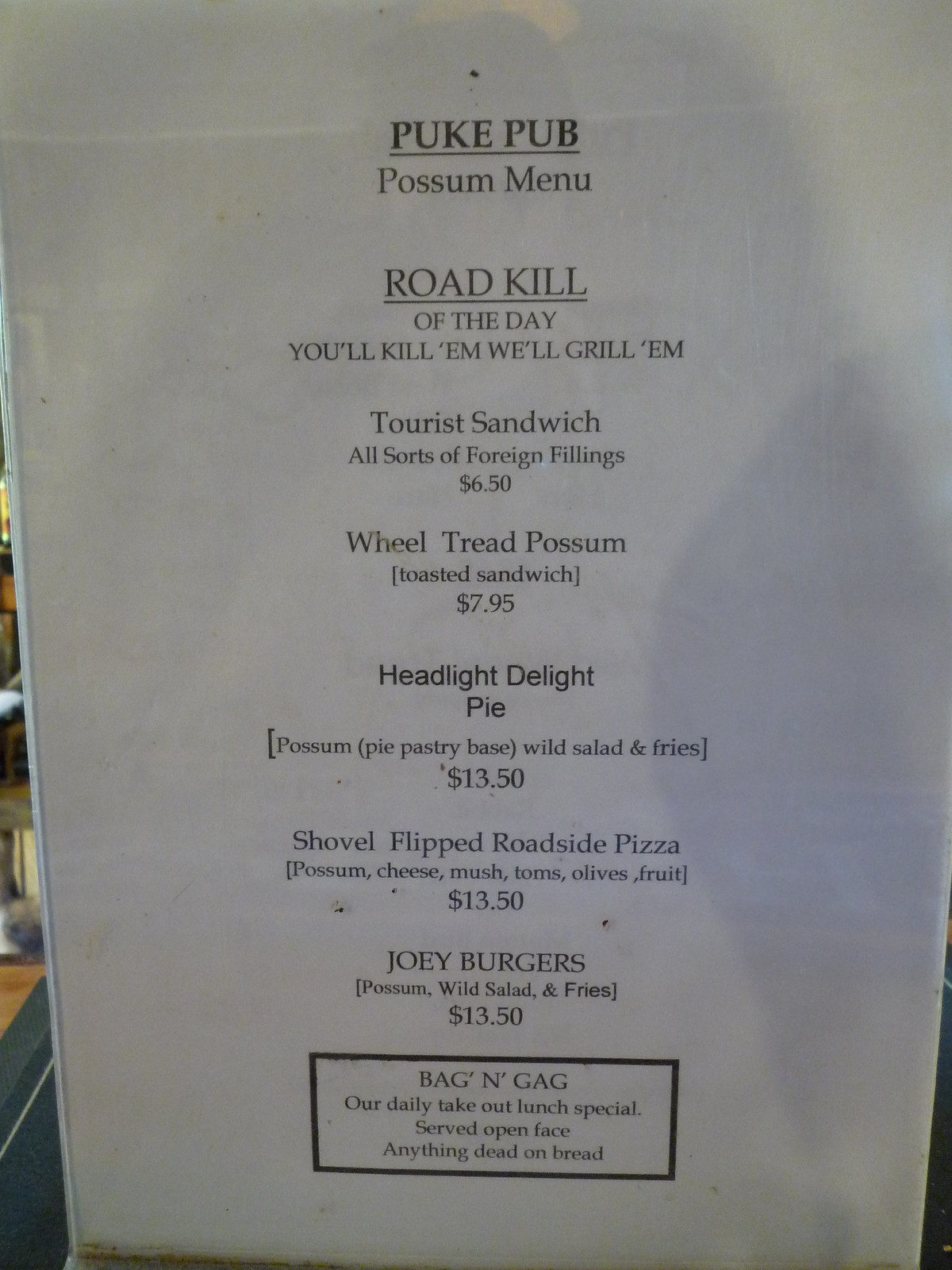The image depicts an off-white sheet of paper displayed within a clear, plastic stand-up sign holder. The sheet is notably thicker than a usual piece of paper, suggesting that it could be laminated or made from cardstock. There is centered, black printed text in a standard font, likely produced by a printer. 

At the top of the menu, the heading "PUKEPUB" is styled in bold, underlined, uppercase letters. Directly below, the subheading reads "POSSUM MENU" in similar formatting. Beneath this, another bold and underlined heading declares "ROADKILL OF THE DAY." Following this, a playful slogan states, "YOU'LL KILL'EM, WE'LL GRILL'EM."

After a noticeable gap, the first item listed is the "TOURIST SANDWICH," described as containing "ALL SORTS OF FOREIGN FILLINGS" and priced at $6.50. Next on the menu is "WHEEL TREAD POSSUM," which is a toasted sandwich priced at $7.95.

The subsequent item is the "HEADLIGHT DELIGHT PIE," described as "POSSUM PIE PASTRY BASE, WILD SALAD AND FRIES," priced at $13.50. The final item listed is the "SHOVEL FLIPPED ROADSIDE PIZZA," which features "POSSUM CHEESE, MUSH, TOMS, OLIVES, FRUIT," and is also priced at $13.50.